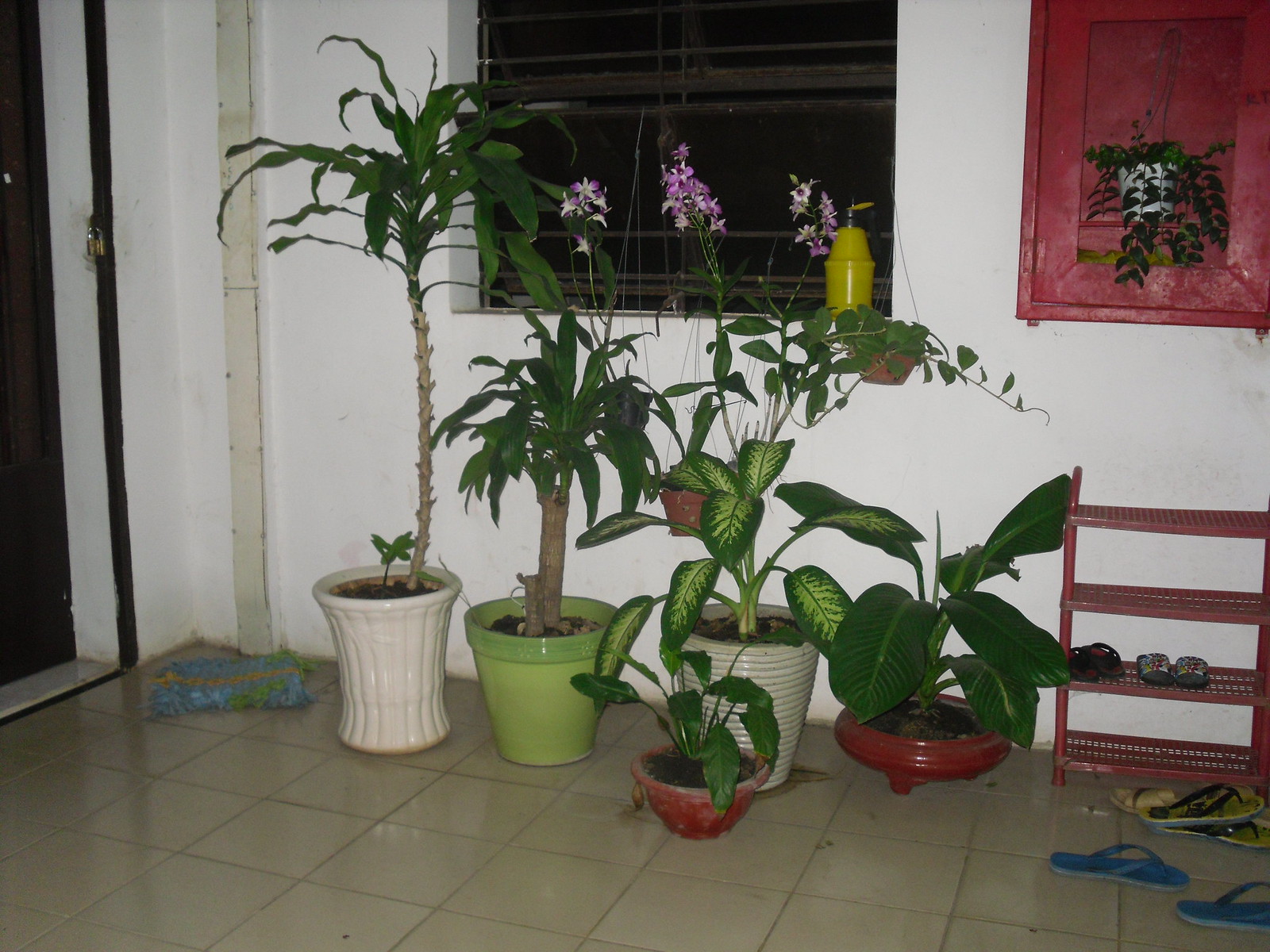This image depicts an indoor area, possibly an entryway or back patio, characterized by a collection of diverse plants and various household elements. The floor is made of reflective beige tiles with grout lines, offering a clean, organized look. Positioned prominently on the left is a tall plant in a large white pot, nearly tree-like in its grandeur. Next to it, several other plants of varying sizes and shapes are housed in distinct pots: another white pot, two red pots, and a lime green one. A few of the plants feature broad green leaves and some even have beautiful lilac blooms.

In the right-hand area of the room, a red plastic shoe rack stands against a white wall, containing two pairs of shoes on the middle rack. Scattered around the shoe rack on the tiled floor are several pairs of flip-flops in blue, green, and neutral beige tones. Adjacent to the shoe rack, a red cabinet is noticeable, featuring a hanging plant with vining greenery cascading from a white pot.

Above the plant display, there is a large window that allows a view into the pitch dark outside. The room also includes a black door with limited visibility and a brown door with possibly broken mini blinds. The walls are predominantly white, with one section tinged with a greenish hue. A folded blue rug lies slightly rumpled on the floor, adding a casual touch to the otherwise orderly space.